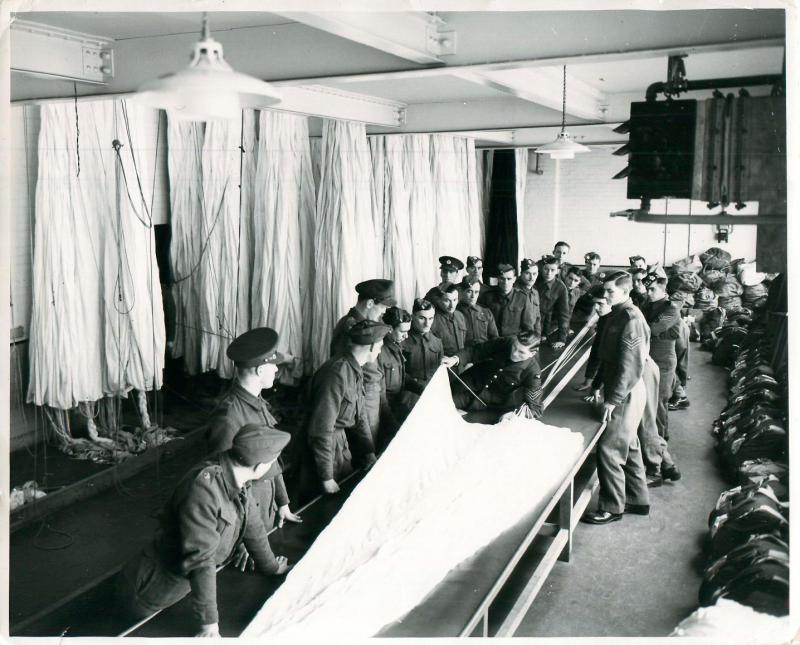In this vintage black-and-white photograph, roughly twenty to twenty-two men in military uniforms with shoulder stripes are gathered closely around a long table. Some uniforms feature pointed caps while others have a rounded dome atop. This detailed scene unfolds in a stark white room adorned with hanging sheets and bags, possibly the men's own property. The men seem to be engaged in an instructional activity, possibly learning to fold a large object or a map, demonstrated by a central figure who appears to be sitting or crouching on the table, giving an impression of floating. The surrounding men watch intently, hands on a long cloth stretched across the table, suggesting they might be assembling or dissembling something. A shelf below the table holds equipment, possibly including an electronic tuner device. The atmosphere is one of focused attention and camaraderie, capturing a moment of military life from days gone by.